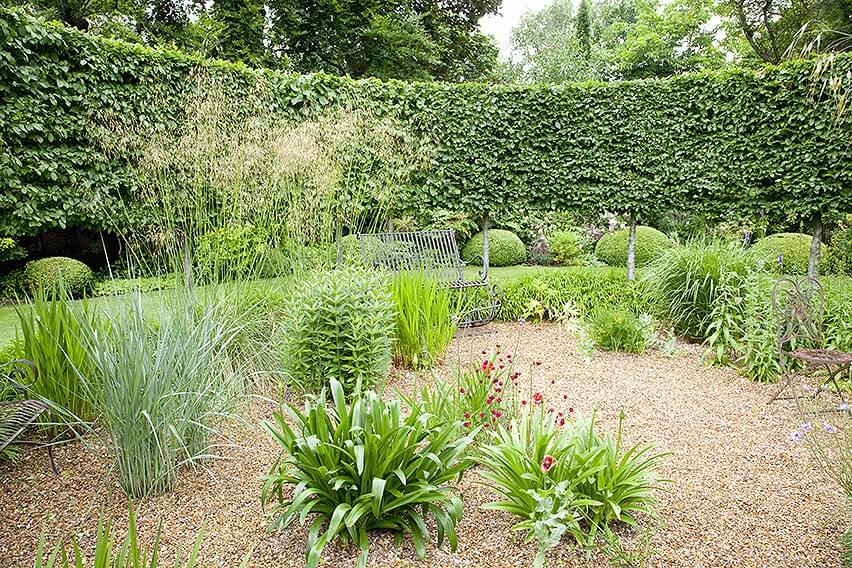The color photograph in landscape orientation captures a meticulously designed garden in a private backyard or courtyard setting. The garden is bordered by a tall, curved hedge that creates a secluded space. In the background, beyond the hedge, tall trees stretch upward. The curved wall backing the garden is covered in ivy, and along its base, perfectly groomed round shrubs are methodically arranged. 

In the foreground, the garden features an irregularly shaped, mulched area with brown pebbles, housing a variety of shrubs and plants, some adorned with red flowers. Scattered throughout this mulched zone, the plants appear randomly yet thoughtfully placed. A wrought iron bench sits towards the back of the garden, offering a resting spot amidst the greenery. To the left bottom section of the image, a lawn sculpture complements the scene. The garden's meticulous design follows the principles of photographic representational realism, emphasizing careful plant positioning and a harmonious arrangement of natural elements. Above, the sky is white, providing a neutral backdrop that enhances the lush greens and vibrant colors of the garden.